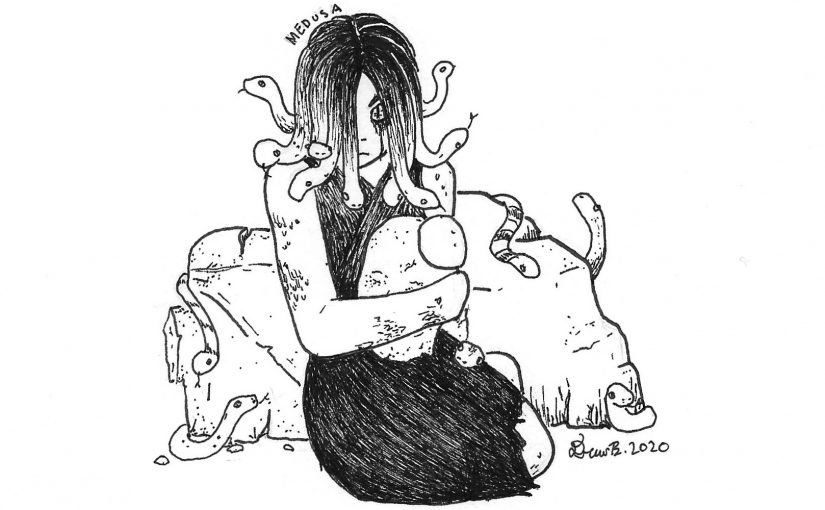The pen drawing shows a woman resembling Medusa sitting on the ground in front of a large boulder. She's wearing a black sleeveless dress that reaches her knees and her hair, which transitions into snakes or slugs at the ends, partially covers her right eye. Above her head, the word "MEDUSA" is written in large black letters. She holds a human head in her hands, her right arm crossing her waist. Her left eye is visible, and she appears to be crying. The boulder behind her is covered with slithering snakes or slugs. In the bottom right corner, the signature "STOP 2020" marks the drawing's completion year. The overall monochromatic palette emphasizes the eerie, mythological theme.